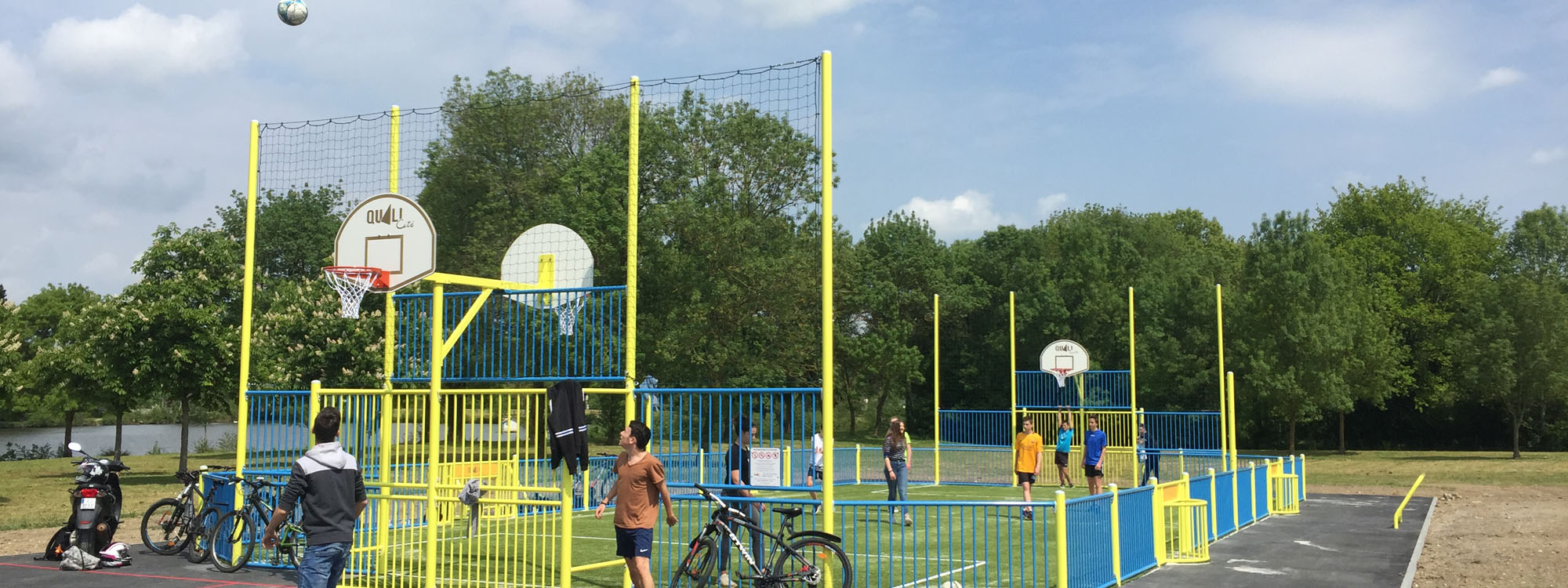This vibrant outdoor photograph captures a lively park on a partly cloudy day, highlighting a recreational area bustling with activity. The sky is dotted with white fluffy clouds, enhancing the fresh, vibrant ambiance. Centered in the image are two basketball courts bordered by yellow and blue fences. The courts are animated by several teenage and preteen boys engrossed in their game. Notably, one basketball is frozen mid-air, having just bounced off a rim, and elicits attention from a few onlookers.

To the left, a four-pole yellow fence with netting and secondary lower fencing is visible, adding structure to the scene. A bike rack, crowded with bicycles and a solitary motorcycle, stands nearby, hinting at the popular transport mode of the young players. The blue and yellow fence continues along the right-hand side, demarcating the rec area from an adjacent gray asphalt surface, which leads into a dirt path and eventually a verdant grove of trees in the background.

Highlighted in the far left of the image is a serene pond, partially obscured by dense greenery. Among the spectators, a man in a jacket and blue jeans faces away, while another individual, clad in shorts and a shirt, is captivated by the ball soaring high above. The mixture of recreational hustle, natural beauty, and dynamic elements captures a quintessential park scene, illustrating a typical day in an outdoor sports haven.